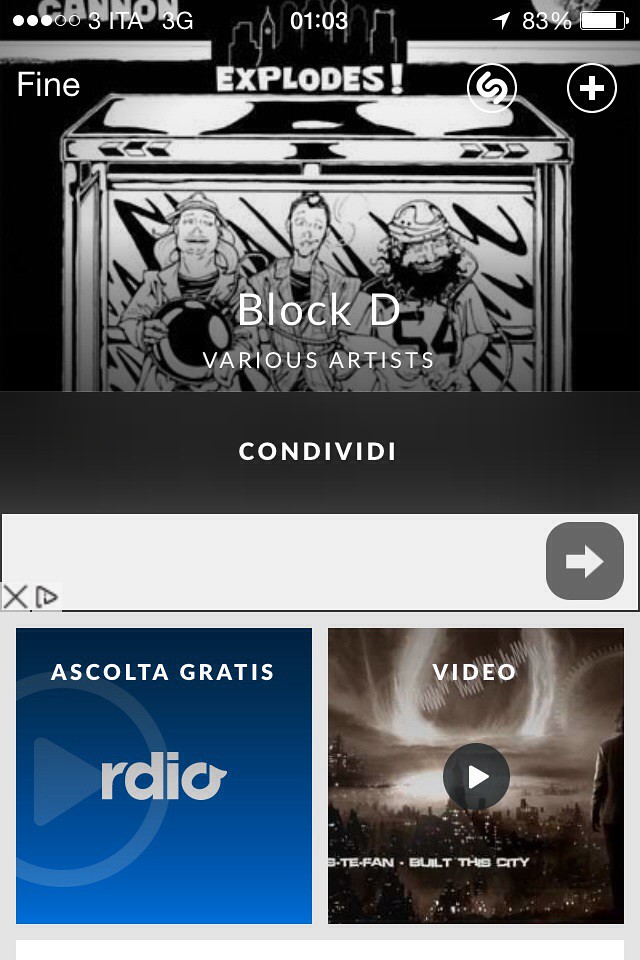The screenshot, taken from a phone, shows a page that strongly suggests the app Shazam. The top of the phone screen indicates a 3G signal with '3ITA3G' on the left, the time as 01:03 in the center, and an 83% battery life on the right. Below, the app interface is divided into distinct sections. The upper half prominently displays an album cover with black and white art depicting three men standing in a cube, labeled "Block D, Various Artists," with the text "Cond Ividy" below it. There are three buttons aligned at the top of this section: 'Find,' a Shazam logo, and a plus sign. Separating the album cover from the content below, there appears to be a blank ad. The lower sections include a blue square on the left stating "Escolta Gratis" with the word "Radio" and another section to the right labeled "Video," featuring an album cover of a gray cityscape illuminated by U-shaped lights and the text "Built This City." These details highlight a multimedia interface, likely used for music identification and streaming.